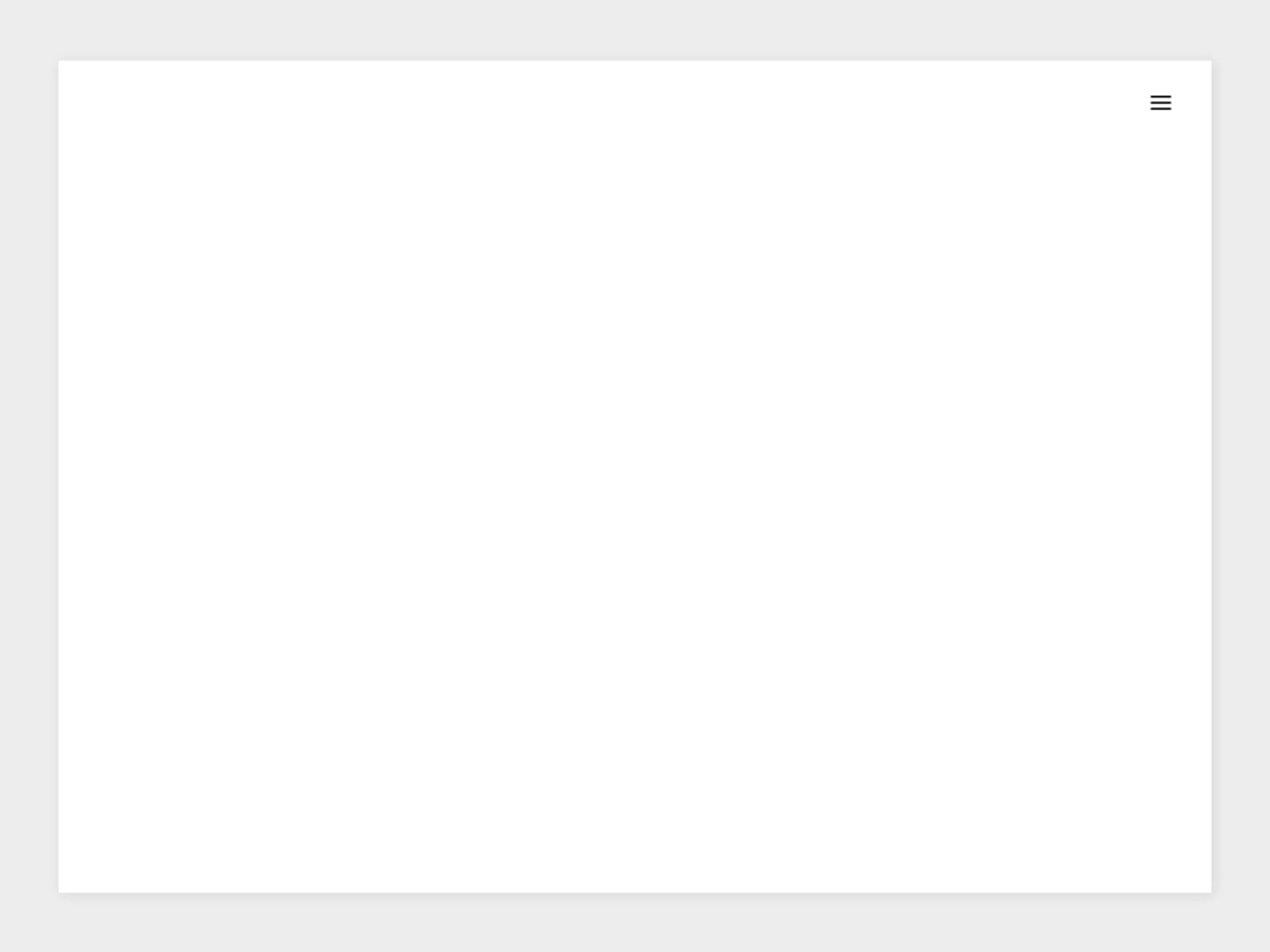The image depicts a minimalistic interface in a landscape layout, most likely from a desktop or a laptop screen, although it could also be a horizontally-oriented tablet. The background is set in a very light grey color, surrounding a central white rectangle, creating a wide border approximately 10 to 12 centimeters in thickness. This white rectangle appears slightly elevated from the grey background due to a subtle shadow effect along its edges. In the top right corner of the white rectangle, there are three small, dark grey or black horizontal lines arranged vertically, one beneath the other, possibly indicating a menu or navigational element.